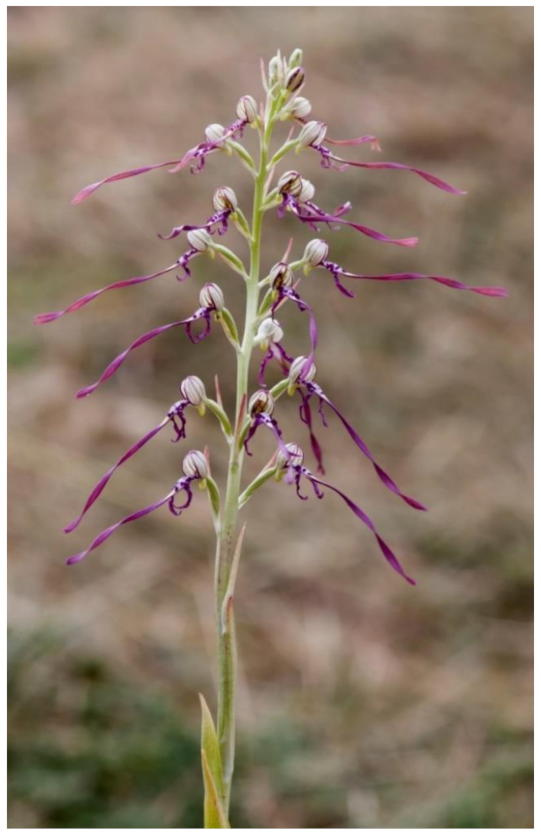This vertical-rectangular image captures a unique wildflower that appears to be in the process of blooming. The focal point of the photo is a tall, slender plant with a green stem extending upwards through the center. From about halfway up the stem, several slender side branches emerge, each tipped with a small, white bulbous structure. From these bulbs, long, vibrant purple streamers cascade downward, accompanied by a few shorter streamers of the same bright violet hue, which subtly transitions to a pink tint towards their ends. The flowers are primarily concentrated at the top of the stem, where a few buds, still in the process of opening, hint at future blossoms. The background features a soft bokeh effect, blending greens and browns—likely representing other plants and bare earth—enhancing the focus on the striking wildflower in the foreground.